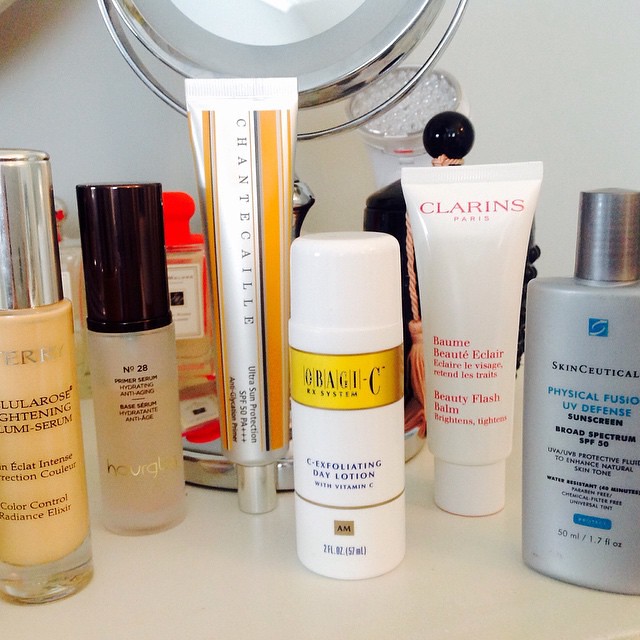A square color photograph, mostly in focus but slightly blurred, showcases a curated collection of high-end cosmetic skincare items arranged neatly on a white surface against a white background. The top part of a chrome-based makeup mirror, which features a two-sided design with one magnifying side, is visible in the background. Beside the mirror, there appears to be an unidentifiable device, possibly a light or facial scrubber.

From left to right, the lineup includes:

1. **Lula Rose Brightening Lumi Serum** - Encased in a clear bottle with a tan-colored liquid and a tall, narrow chrome screw-on cap.
2. **Number 28 Serum** - Housed in a frosted bottle with a sleek, tall black cap. The label is unreadable.
3. **Background Perfume Bottles** - These square bottles with screw-on caps resemble eau de toilette containers.
4. **Chantecaille Sun Protection SPF 50** - A luxurious sunscreen in a white tube featuring orange and gray stripes, standing upright on its screw-top.
5. **Obagi C Exfoliating Day Lotion (AM)** - Appears to be a roll-on deodorant but is actually a premium white lotion bottle labeled "Obagi C," with a 2-ounce capacity.
6. **Clarins Paris Beauty Flash Balm** - This is a white squeeze tube labeled "Eclat Minute," a brightening lotion designed to enhance radiance.
7. **SkinCeuticals Physical Fusion UV Defense Sunscreen SPF 50** - Presented in a distinctive blue bottle with a gray screw-on cap.

This array of skincare and cosmetic products likely amounts to several hundred dollars, emphasizing the high quality and luxury of the items.